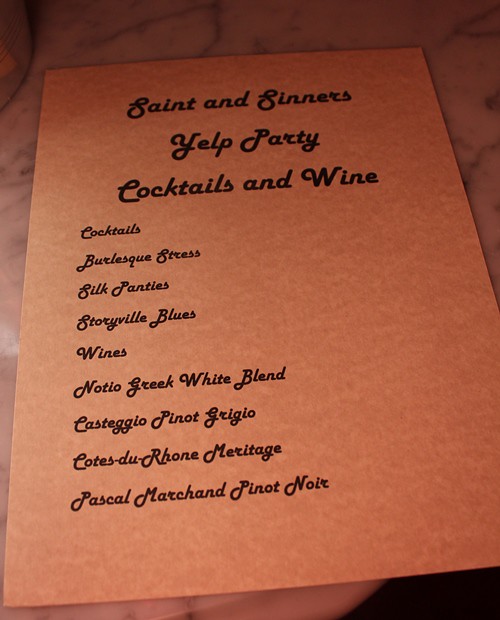The image is a vertically aligned rectangular photograph of a menu lying on a marbled countertop with white and gray swirls. The menu appears to be made of brown cardboard and has black text printed on it in a cursive, curly-based font. At the top, centered, it reads "Saint and Sinners Yelp Party Cocktails and Wine." Below this, left-aligned, is a list in smaller cursive font detailing cocktails and wines. The cocktail section includes "Burlesque Stress," "Silk Panties," and "Storyville Blues." The wines listed are "Notio Greek White Blend," "Castegio Pinot Grigio," "Cote du Rhone Meritage," and "Pascal Marchand Pinot Noir." The entire image is somewhat dark, with a light maroon shade overall.